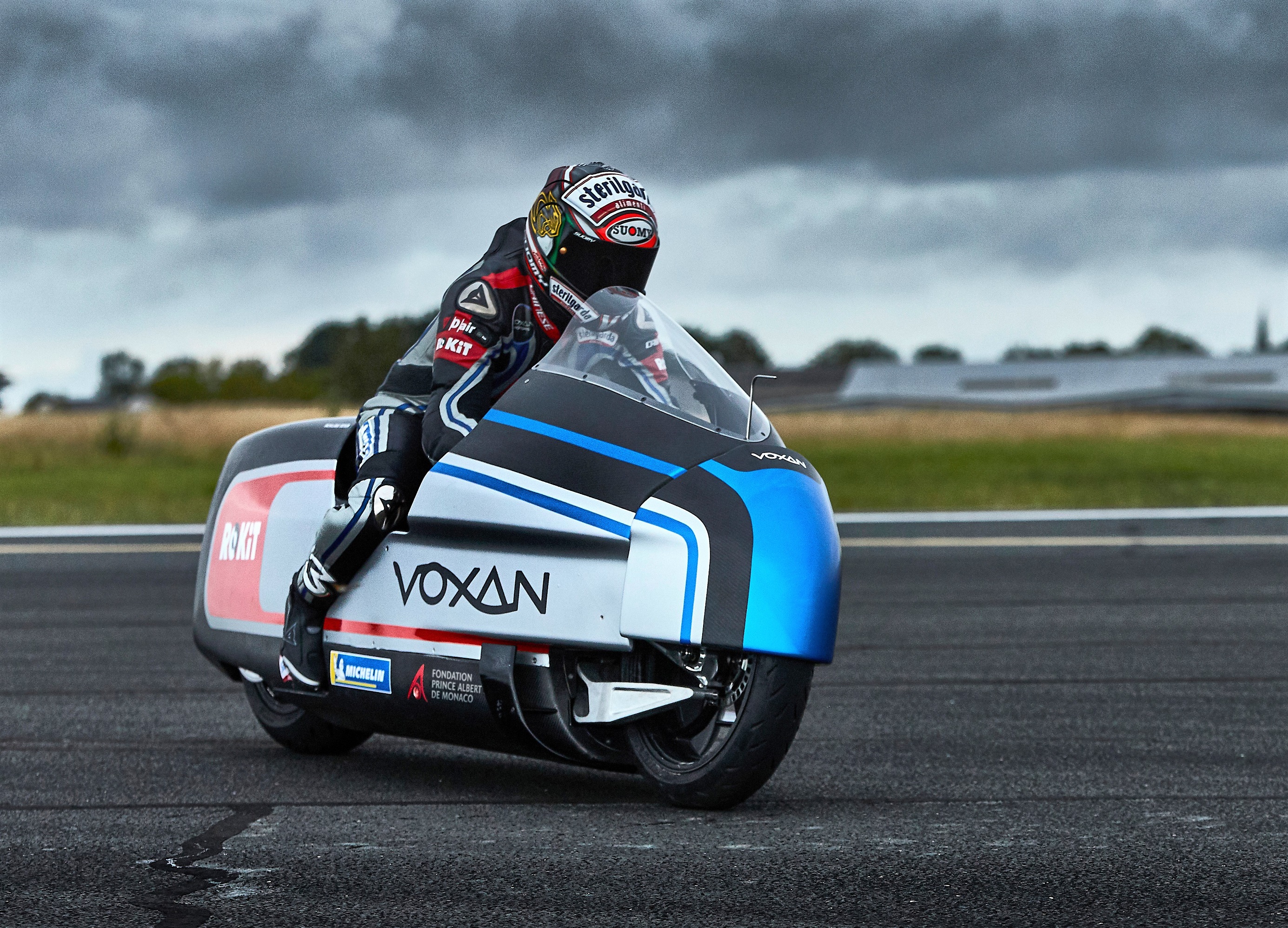This outdoor photograph captures an intense moment of a motorcyclist speeding on an asphalt road under a brooding, stormy sky with dark, gray clouds. The rider is mounted on a sleek and contemporary motorcycle, predominantly white with stylish, rounded edges that enhance its aerodynamic design. The motorcycle is emblazoned with the name "Voxan" in black lettering on its silver side and front, while "Foundation Prince Albert de Monaco" is written between its wheels. The vehicle's smooth, boxy form features a unique blue tip and the wheels are stark black.

The motorcyclist is clad from head to toe in a black riding suit adorned with numerous sponsor logos, including a helmet with a distinctive black-tinted visor and an array of sponsor texts and logos, one of which reads "Stereo Ligger" on a white strip at the top. The rider’s face is fully obscured by the helmet, adding to the sense of speed and anonymity. Behind the motorcyclist, the blurred background reveals fields and a nondescript, grayish building, emphasizing the focus on the rider and the high-performance motorcycle cutting through the dismal weather.